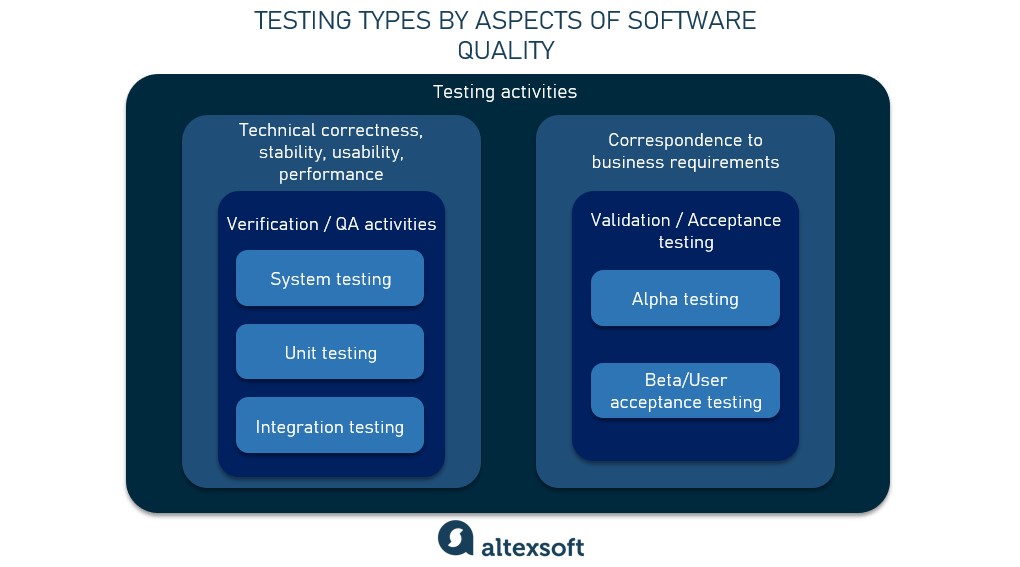The image is a color illustration infographic in landscape orientation titled "Testing Types by Aspects of Software Quality" in dark blue, all caps, centered at the top. Below this title, there is a dark blue horizontal rectangle with rounded corners labeled "Testing Activities" in white text. The infographic is divided into two main sections, represented by portrait-oriented medium blue rectangles side-by-side.

The left section is titled "Technical Correctness, Stability, Usability, Performance" in white text. Underneath, a darker blue vertical rectangle with rounded corners is labeled "Verification / QA Activities" (Quality Assurance) in white. Within this dark blue rectangle, there are three smaller blue boxes labeled "System Testing," "Unit Testing," and "Integration Testing."

The right section is titled "Correspondence to Business Requirements" in white text. Below this, a darker blue vertical rectangle with rounded corners is labeled "Validation and Acceptance Testing" in white. Within this rectangle, there are two lighter blue boxes labeled "Alpha Testing" and "Beta (User Acceptance) Testing."

At the bottom of the infographic, the logo "Alltechsoft" is displayed. The logo features an S inside a conversation balloon; the S is white, and the balloon is dark blue.

The overall design is characterized by the use of blue shades and rounded corners for all boxes, providing a clean and structured presentation of different testing types related to software quality.